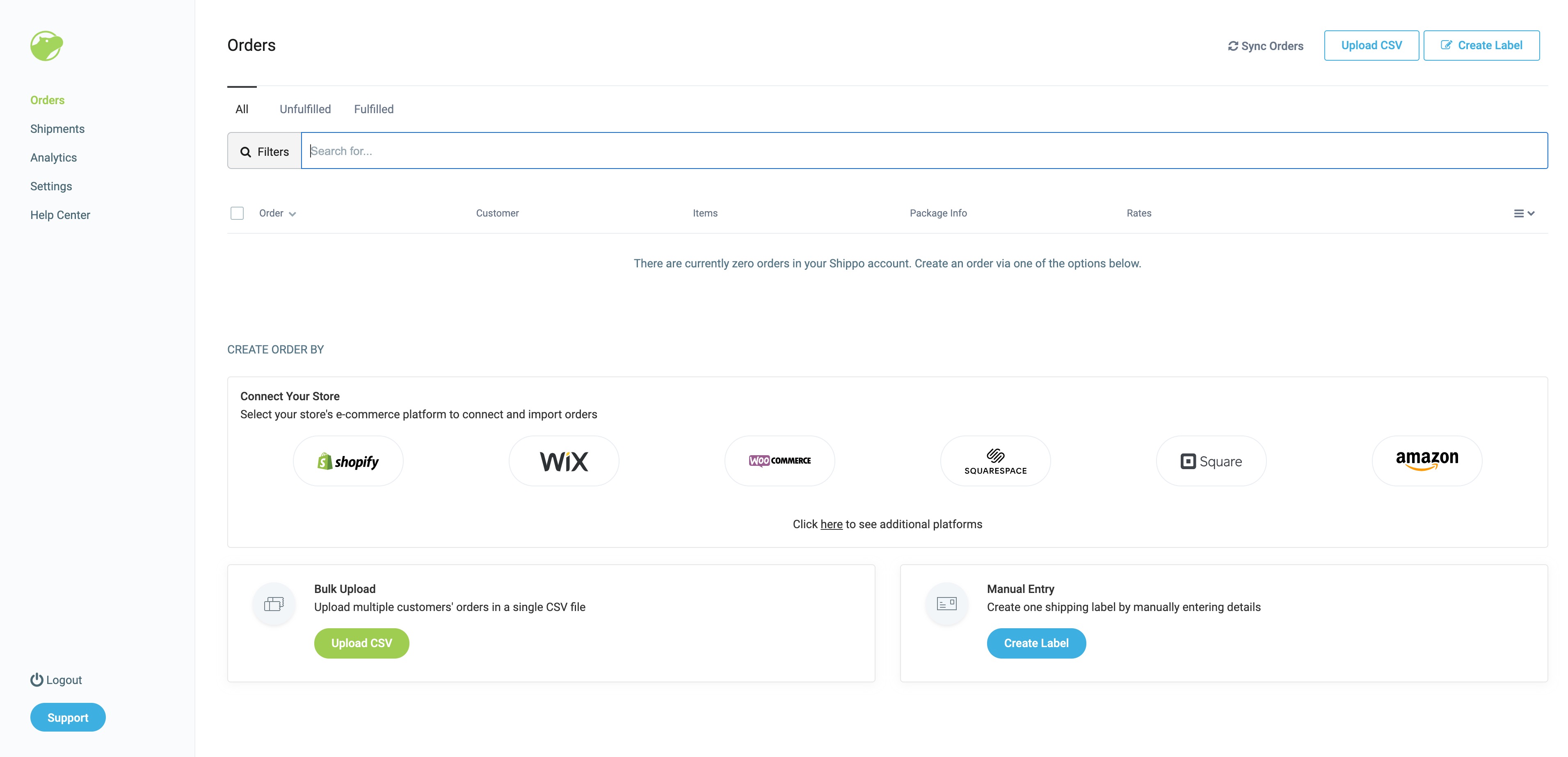The image is a wide rectangular screenshot of an order page from an online store interface, presumably related to multiple e-commerce platforms. At the bottom, there is a highlighted section with the text "Create, Order, Buy," followed by a selected or input dataset indicating connectivity with Shopify. Adjacent to the Shopify reference, the text "W-I-X" or "W/X" is visible, signifying another integrated platform.

Further to the right, icons representing Amazon and Squarespace are visible. Another icon is also present, though its text remains unreadable. Below this section, there is an option for "Bulk Upload" with explanatory text stating, "Upload multiple customers' orders in a single CSV file." 

Following this is a pair of buttons colored red and green designed for uploading. To the right of this setup is a separate window titled "Manual Entry," accompanied by a brief sentence, "Create one shipping label by manually entering details." Underneath this description is a small blue button labeled "Create Label."

This detailed interface illustration captures the essence of the online store's multi-platform integration and functionalities, highlighting options for bulk uploads and manual shipping label creation.